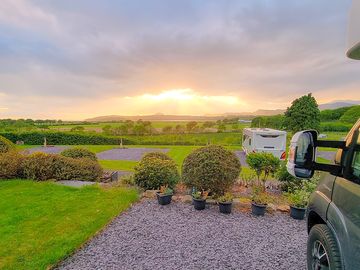This detailed photograph captures a well-maintained outdoor park or campground area characterized by lush, green grassy fields, trimmed bushes, and neatly lined plots of potted plants. The scene is dominated by a cloudy sky with the sun peeking through, casting an orange hue on the horizon as it sets. In the right corner of the image, a dark green vehicle is partially visible, showcasing only its front driver's side, including the side panel, rearview mirror, and front tire. Central to the composition is a white camper trailer parked on a gravel driveway, which stretches out in various directions. The landscape extends out up to two or three miles, encompassing grassy hills and gravel-covered lots, all nestled within the expansive greenery of the campground setting.